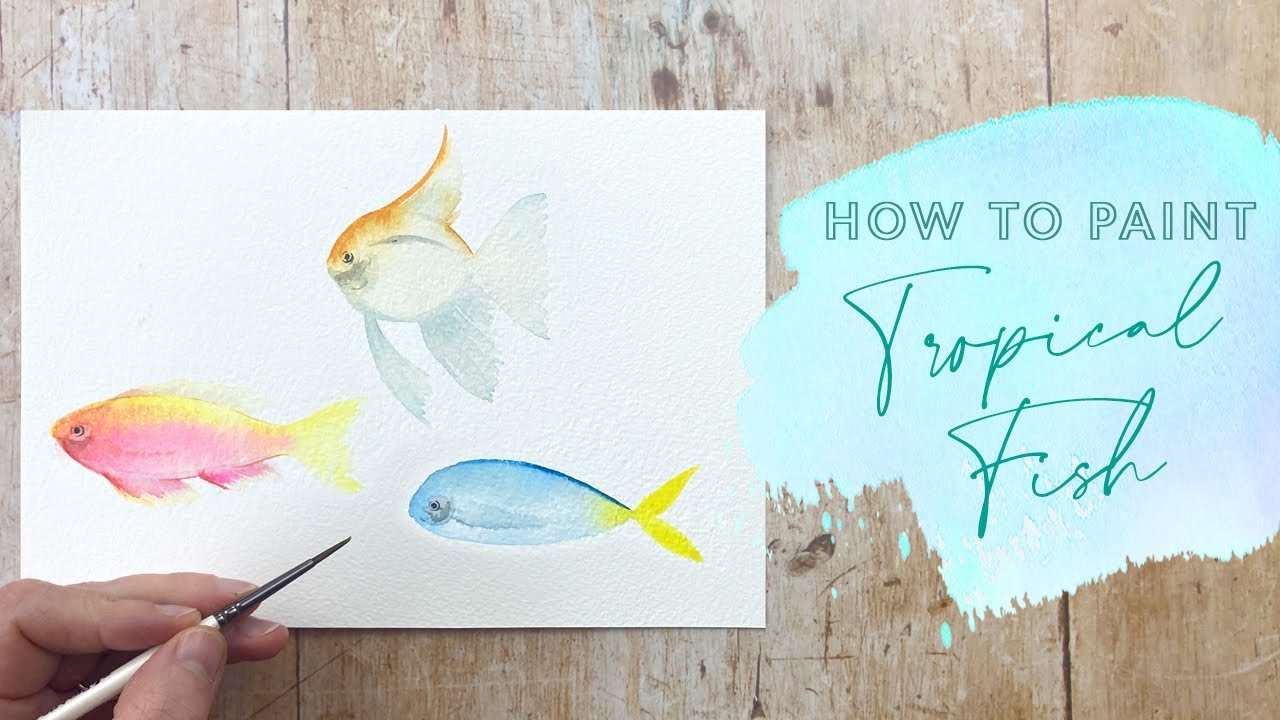The image depicts a wooden background composed of vertically arranged light brown slats. On the right side of the wooden backdrop, there is a section that appears to be haphazardly painted with teal. Overlaying this teal paint are the words "how to paint" in hollow grey text, and the phrase "tropical fish" in a cursive, darker teal or lighter green font. 

On the left side of the image, a piece of white textured paper or canvas is placed against the wooden background. This canvas features three watercolor fish paintings: the fish at the bottom right is predominantly light blue with a dark blue top and a yellow tail; the fish at the top is gold with a white belly and blue fins and gills; the fish on the far left is pink on the bottom and yellow on top. A hand, positioned in the bottom left corner, is holding a white-handled brush with a metallic tip and a dark, almost black bristle, presumably continuing to paint the fish on the canvas. The image combines photographic realism with digital editing to enhance the details and text, giving it a dynamic, creative feel.